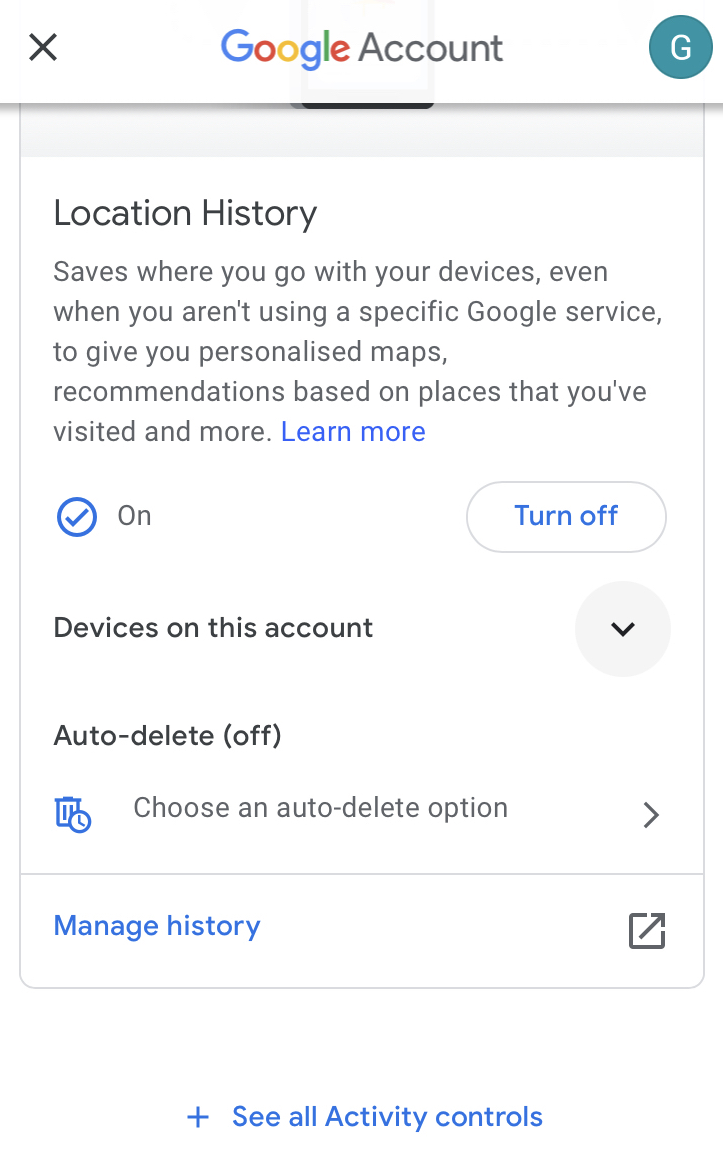This is a detailed caption for an image of a Google settings screenshot:

---

This image captures a screenshot of Google's account settings, specifically focusing on the location history section. The photo is in portrait orientation with a white background, although it lacks clearly defined borders. At the top of the screen, the banner reads "Google Account" in a white strip with the word "Google" rendered in its iconic color scheme: blue, red, yellow, blue, green, and red. To the left of the banner, there's a black "X" (presumably for closing the window), and to the right, a green circle containing a white "G," likely indicating a user profile or avatar.

Beneath the header, the section transitions from a gray box, partially covered by the transparent "Google Account" text, to a white area. The main focus is "Location History," which is followed by an explanation stating, "Saves where you go with your devices, even when you aren’t using a specific Google service, to give you personalized maps, recommendations based off places you've visited more." A "Learn more" link is also provided.

Below this explanation is a blue checkmark within a white circle, indicating the option is enabled. Next to it, a blue circle with the word "On" further confirms the status. Adjacent to this is a button with a gray border, white interior, and blue text that reads "Turn off."

Further down, a heading in black text states, "Devices on this account," followed by a gray box featuring a black checkmark. Inside the box, the status "Auto-delete off" is printed in black. An icon of a garbage can lies underneath, with text prompting users to "Choose an auto-delete option."

At the bottom, a blue hyperlink reading "Manage history" is followed by an "Open" button. Outside of this box, a blue plus sign accompanied by the text "See all activity" is visible, indicating more options are available.

---

This descriptive caption provides a thorough and structured visual depiction of the content within the screenshot of the Google account settings.